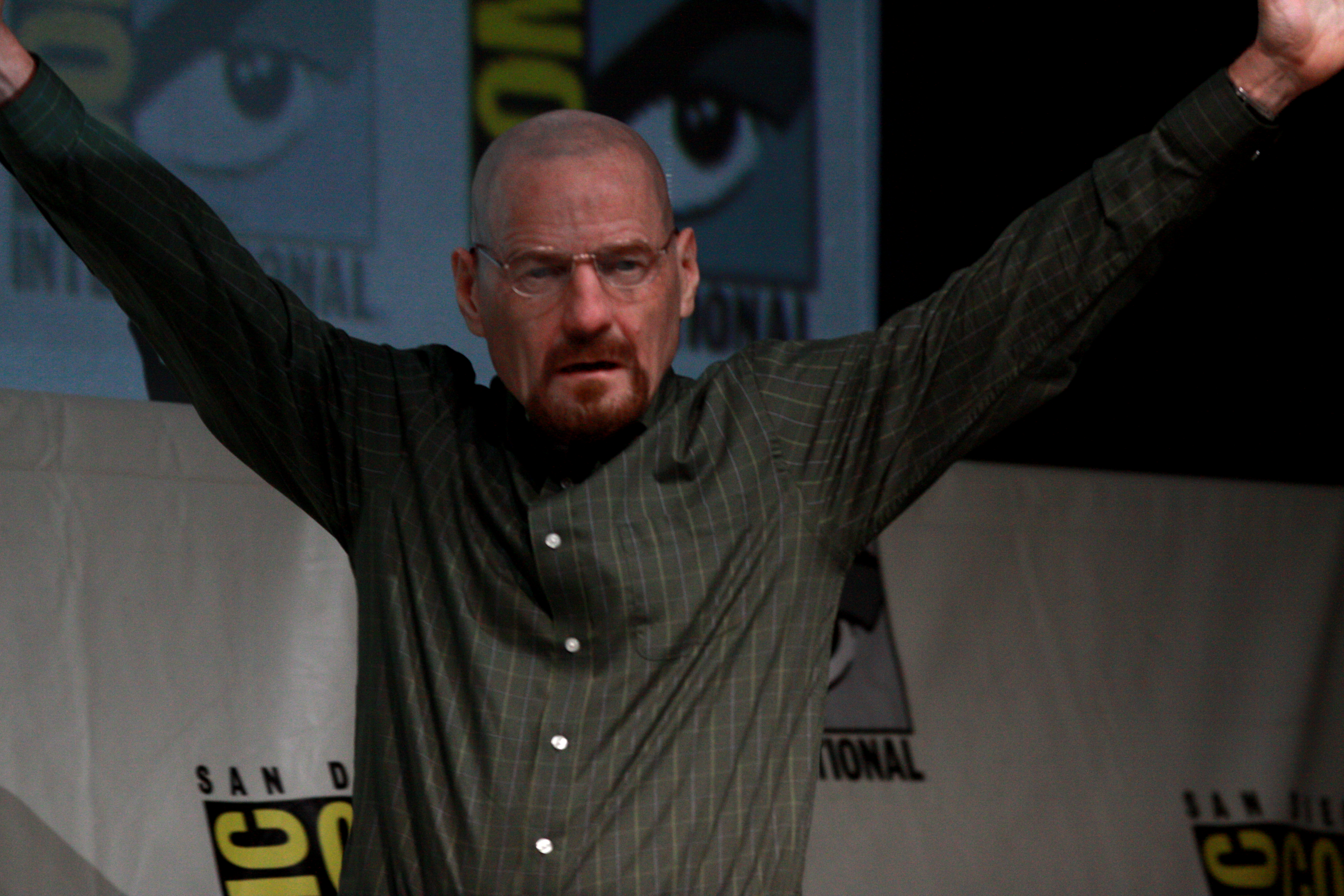This image captures Bryan Cranston, famously known for his roles in "Breaking Bad" and "Malcolm in the Middle," at San Diego Comic-Con. Cranston is dressed as his iconic character, Walter White, complete with a bald head, glasses, and a reddish goatee. He sports a gray, long-sleeved, collared shirt with buttons down the middle and a watch on his left wrist. His arms are raised in a V shape, and he stands under a spotlight on stage. The background features a repeating white backdrop with the San Diego Comic-Con logo and partial images of an anime character's eyes. There are also segments of text in yellow and black, partially obscured by his pose.